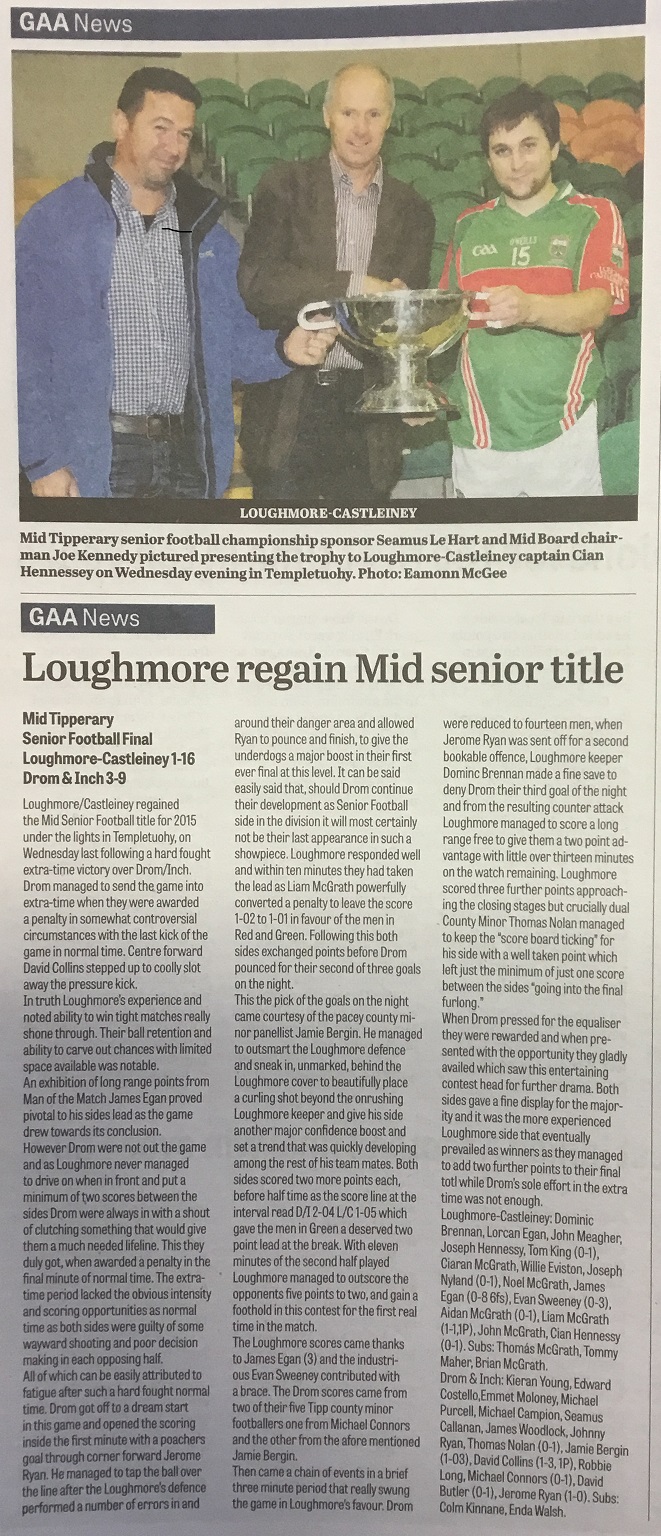In the image, a newspaper article from the GAA News section is displayed, topped with a photograph and followed by a detailed written article. The photograph depicts three men standing in a sports venue, likely a stadium, with a background of green seats. 

The man on the left is dressed in a blue jacket over a checkered shirt. The man in the middle wears a brown blazer over a light-striped shirt, while the man on the right sports a green and red jersey with the number 15 and the letters "GAA," indicating one of the sponsors.

The man in the middle is holding a large silver trophy, which the other two men are touching. Below the photograph, the caption reads: "Mid-Tipperary Senior Football Championship Sponsor Seamus Lehart and Mid-Board Chairman Joe Kennedy presenting the trophy to Laumore Castellini Captain Cian Hennessy on Wednesday evening in Templetuohy. Photo by Emman McGee."

The article is titled "Laumore Regain Mid-Senior Title" in bold. It details the Mid-Tipperary Senior Football Final, where Laumore Castellini triumphed over Drom and Inch with a score of 1-16 to 3-9 in a hard-fought, extra-time victory. Although the text is small and hard to read, the article provides a comprehensive recap of the match, celebrating Laumore's victory and highlighting key moments and player performances.